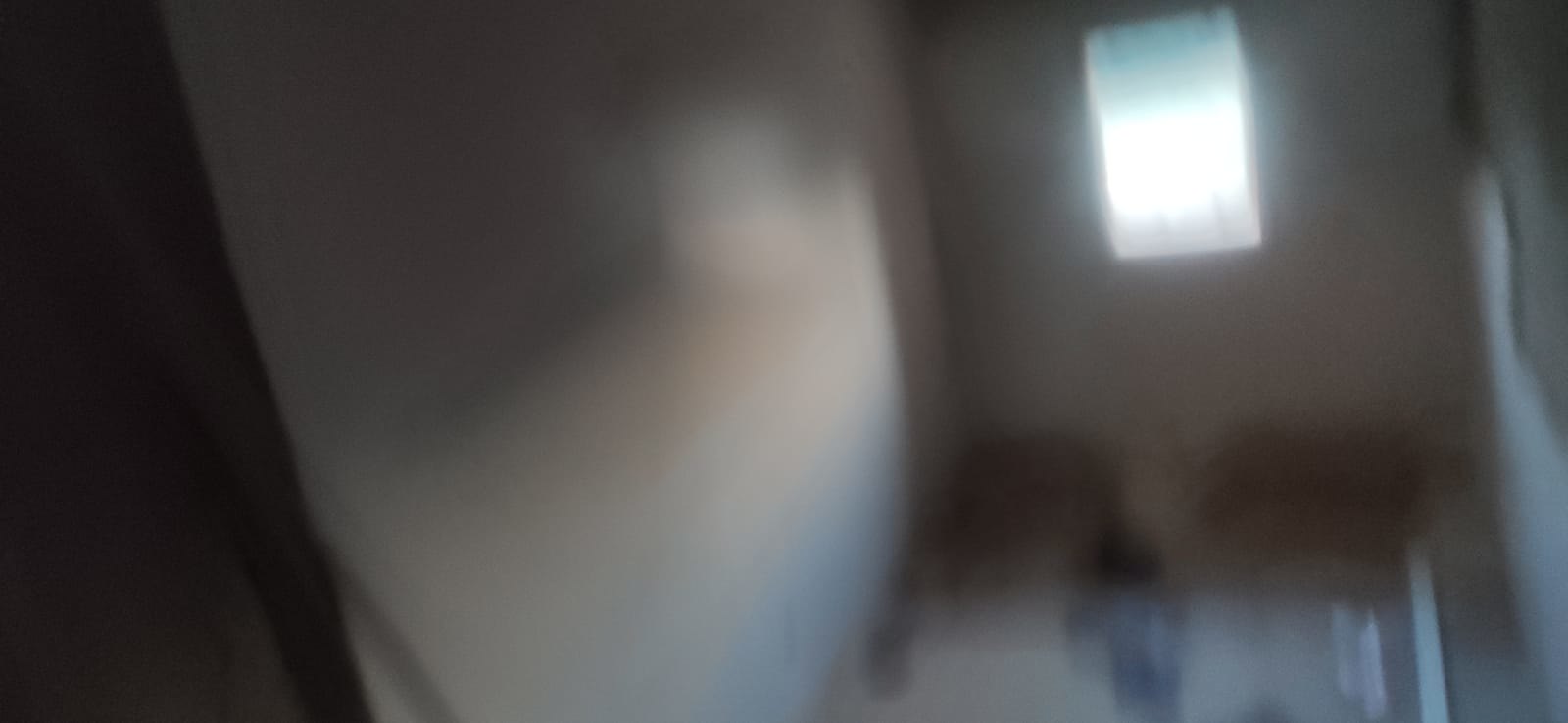The image depicts a somewhat blurry indoor photo of a narrow, elongated nook. The walls, painted an off-white color, form a confined space approximately the width of three standard rectangular windows. A window is situated at the far end on the right side of the photo, allowing some natural light into the dim passage. To the left, the wall appears to curve, suggesting the nook might lead into a cellar-like or rounded area, though this part remains unclear due to the photo's angle and blurriness. The floor of the space appears unfinished, adding to the overall sense of an undeveloped setting. The camera seems to be held at a slight angle, diagonally towards the upper left, adding to the disorienting feel of the scene.